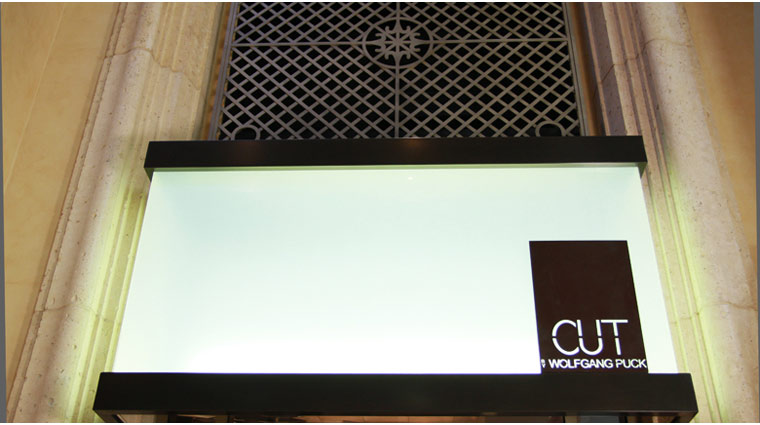The image captures an indoor setting within a decently fancy building. Prominently featured at the bottom center of the image is a rectangular object, primarily white with a black top and bottom, resting against a light beige tiled wall adorned with columns on either side. This object appears to be a package or possibly a sign mounted on the wall. In the bottom right corner of this object, the text "cut Wolfgang Puck" is clearly visible in white letters on a black background. Above the rectangular object, a window framed by a metal mesh or ventilation system is situated, adding to the image's well-lit and clear appearance, thanks to abundant natural light. The elegant combination of tan, white, brown, black, gold, and cream colors further enhances the sophisticated ambiance of the setting.